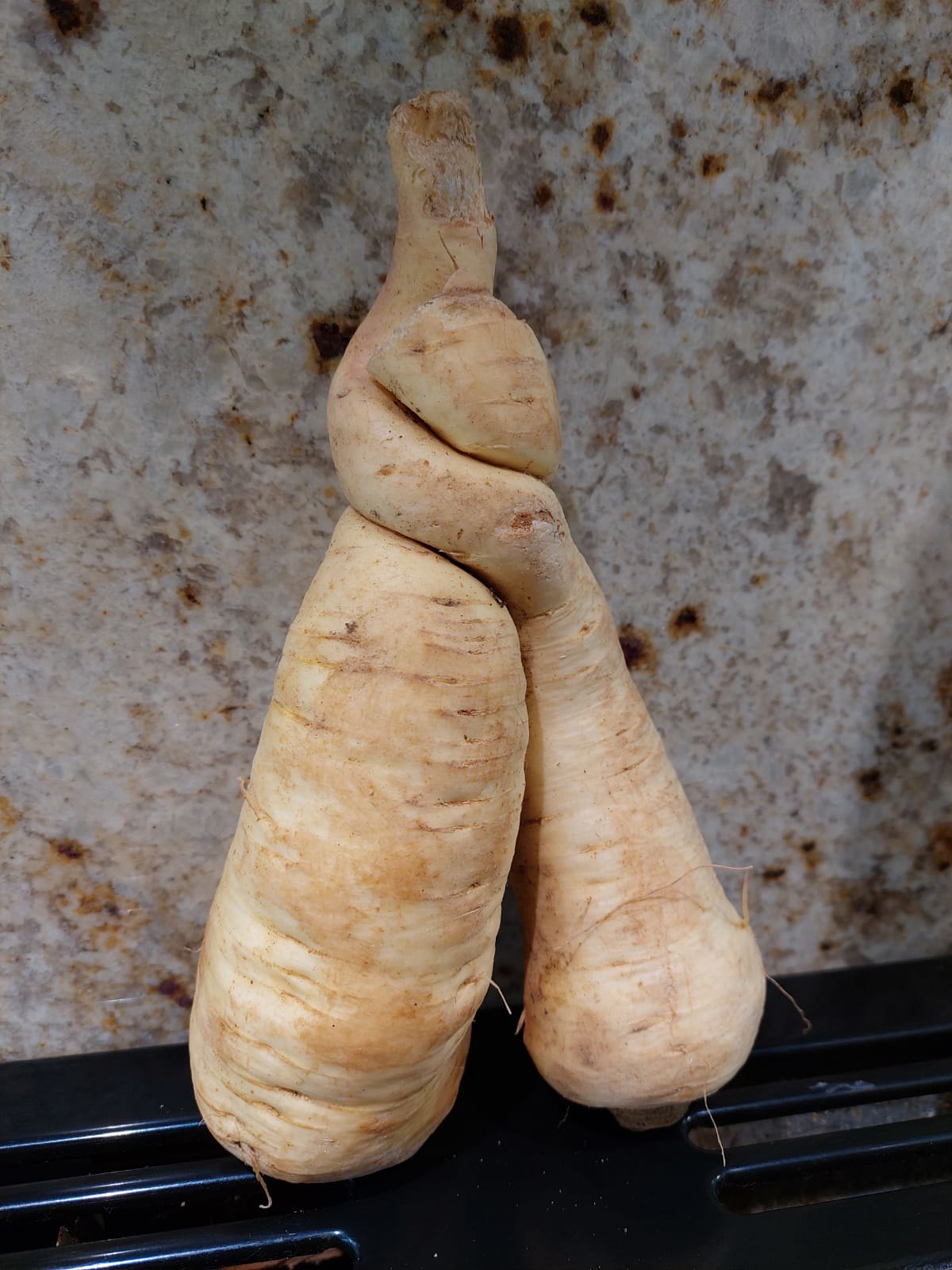This photograph showcases two intertwined radishes, conjoined at their tail ends, evoking the appearance of embracing each other. They lean against a stone-like, grayish light brown marble textured backdrop, standing upright on a dark blue metallic surface with wide slits. The radishes exhibit a gradient of colors, starting from a light yellow to orangish hue, with notable brown shades and several roots sprouting from them. No text is present in the image.  In the background, a wad of white material speckled with brown spots adds an additional layer of visual interest. The image, likely taken indoors, emphasizes the roots or produce as its focal point, highlighting their unique intertwined form.